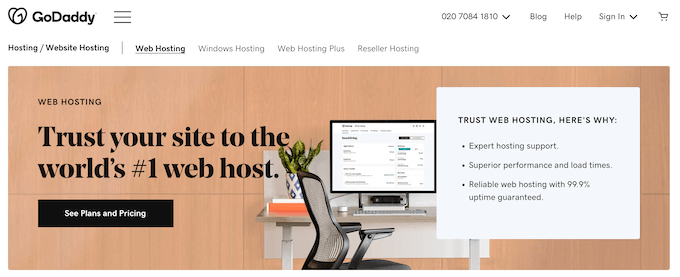In this image, the top left corner features the "GoDaddy" logo in black text, denoting the name of the page. To the right of this logo, there is a menu icon, and further to the right, there are drop-down menus and several textual items including a contact number "020708418110", alongside "Blog", "Help", "Sign In", and an icon of a cat. The background across the top section is white, with all text elements displayed in black.

Directly beneath the "GoDaddy" logo on the left side, there are several tabs listed: "Hosting" or "Website Hosting", "Web Hosting", "Windows Hosting", "Web Hosting Plus", and "Reseller Hosting". These tabs are also in black text against a white background. 

Lower on the page, occupying the main content area, the background filter shifts to brown, while the text remains black. On the left side, it reads "Web Hosting, trust your site to the world’s number one web host." Below this is a prominent black button with white text that states "See Plans and Pricing."

On the right side of the main content area, the text outlines the benefits of their web hosting services: "Trust Web Hosting, Here is Why: Expert Hosting Support, Superior Performance and Load Times, Reliable Web Hosting with 99% Uptime Guaranteed."

Centrally placed within this section is an image of a laptop on a table accompanied by a chair and decor elements. The laptop is situated on a table that has a slight white tint, the keyboard is on the table, and a code plant in white and blue is visible. The plant itself is green, and the chair next to the table is black.